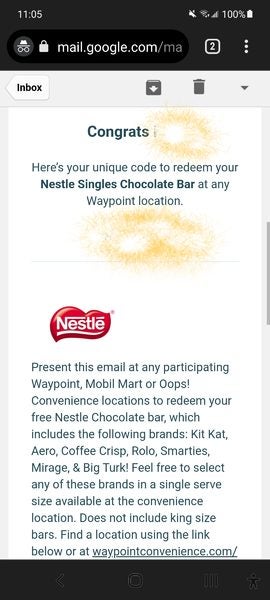The image depicts a cell phone screen with the time displayed as 11:05 AM and a fully charged battery at 100%. The notification bar indicates that the sound is muted. The web browser is open to "mail.google.com," as shown in the search box. There are two open tabs, and the current one displays an email with the subject "Congrats! Here's your unique code to redeem your Nestle single chocolate bar at any Waypoint location."

The email interface shows familiar icons like a trash can for deleting messages and a download arrow for attachments. The email body has a distinctive red symbol with white text reading "Nestlé."

The email announces that the recipient can present the email at participating Waypoint, Mobile Mart, or OOPS convenience locations to redeem a free Nestlé chocolate bar. The offer is valid for various single-serving chocolate brands, including KitKat, Aero, Coffee Crisp, Rolo, Smarties, Mirage, and Big Turk. It specifically excludes king-size bars. The email provides an option to find a store location via a link labeled "waypointconvenience.com."